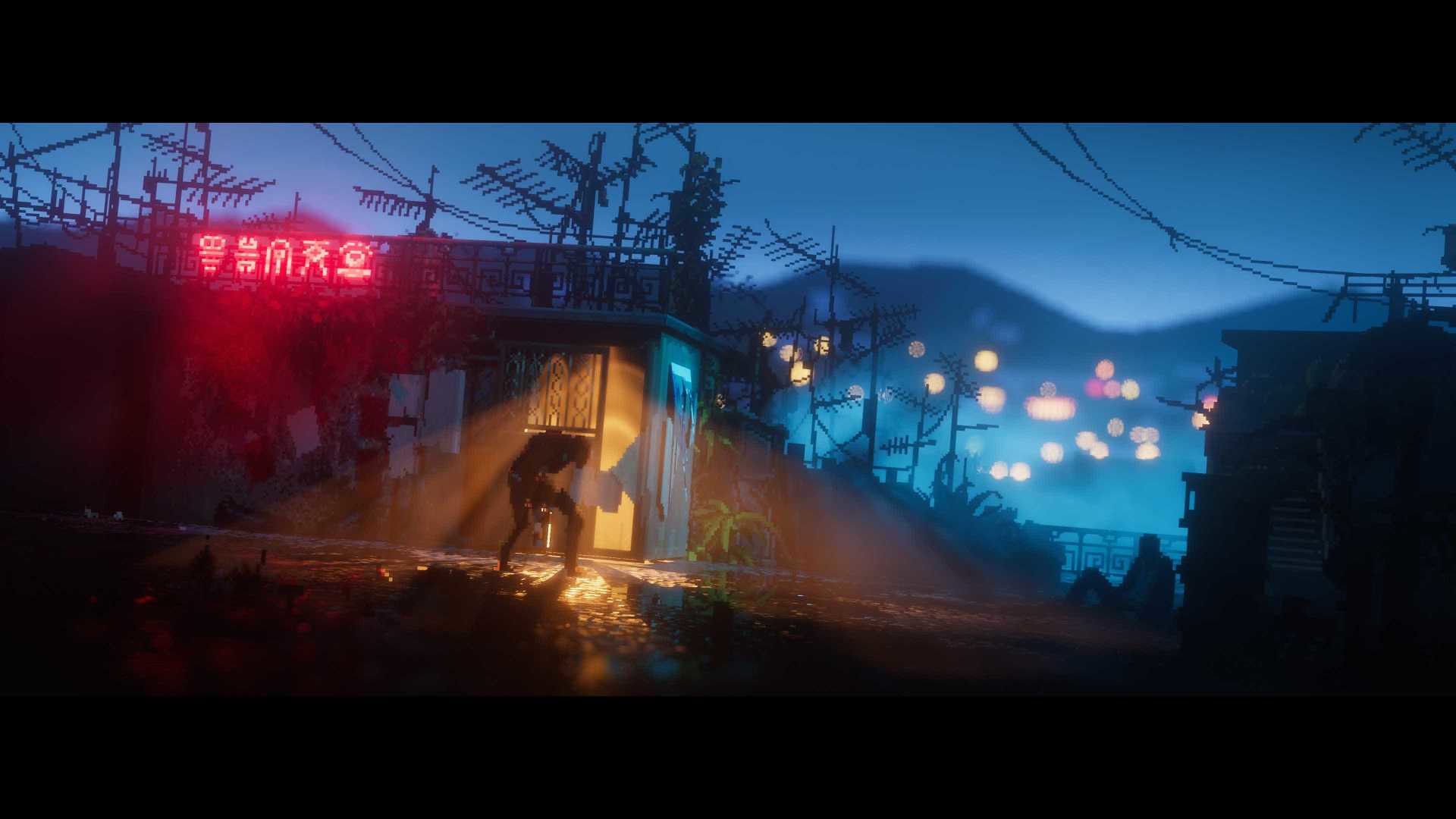In this image, we're presented with a scene from a video game set in an outdoor environment. The composition features a stark contrast with black backgrounds at both the top and bottom. Central to the image is a character, depicted in dark brown and positioned at a considerable distance, appearing as a shadowy silhouette. The character is hunched over, leaning to the right. Directly behind this figure stands a small structure, adorned with five glowing red characters in what appears to be an Asian script, situated at the top of a railing.

To the right of the central character, another silhouette is visible, giving the impression of an individual seated with one knee raised. Further to the right, the edge of another building is seen, accompanied by power lines extending from the top. The background showcases a gradient of light blue hues interspersed with periodic white circular lights, resembling a hill-like formation leading up to a pale blue sky. The overall atmosphere of the scene is serene yet enigmatic, invoking curiosity about the narrative unfolding in this digital landscape.